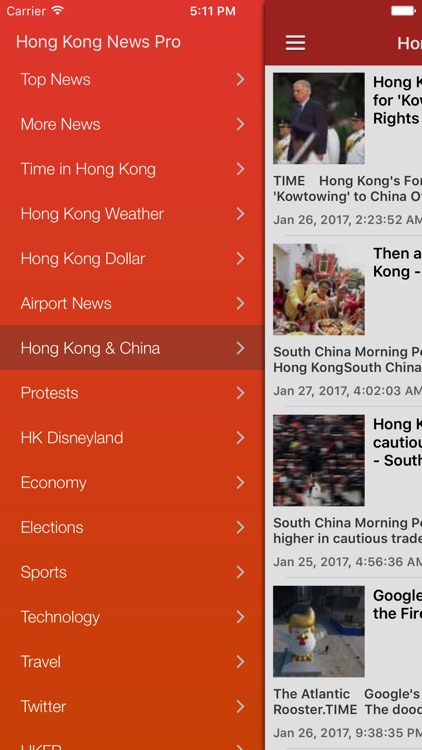This screenshot captures the interface of a news website, specifically titled "Hong Kong News Pro," displayed against an orange backdrop. At the top, the interface indicates the current time as 5:11 PM, displays a Wi-Fi symbol, and includes the word "carrier," suggesting mobile web access. Down the page, beneath the main title, a series of submenus are available with expandable options, marked by small pull-down arrows. The submenus listed are: "Top News," "More News," "Time in Hong Kong," "Hong Kong Weather," "Hong Kong Dollar," "Airport News," and "Hong Kong and China," the latter highlighted within a burgundy box.

Following the submenus, additional categories such as "Protest," "HQ," "Disneyland," "Economy," "Elections," "Sports," "Technology," "Travel," and a partially visible "Twitter Liked," continue. On the right side of the screenshot, a red banner with white accents leads to visible icons and a battery status indicator.

The section below the banner includes several news headlines and associated photographs. The first headline, partially obscured, pertains to rights in Hong Kong, dated January 26, 2017, accompanied by an image of a man with gray hair in a suit. The next headline mentions the "South China Morning," dated January 27, 2017, featuring a picture of people dressed in yellow, seemingly in a celebratory frame. Below this, a blurry photograph accompanies a headline on cautious trading in the "South China Morning," dated January 25, 2017. The final visible headline relates to "Google's rooster time" from "The Atlantic," showcasing a quirky white character with an orange beak and yellow hair, dated January 26, 2017.